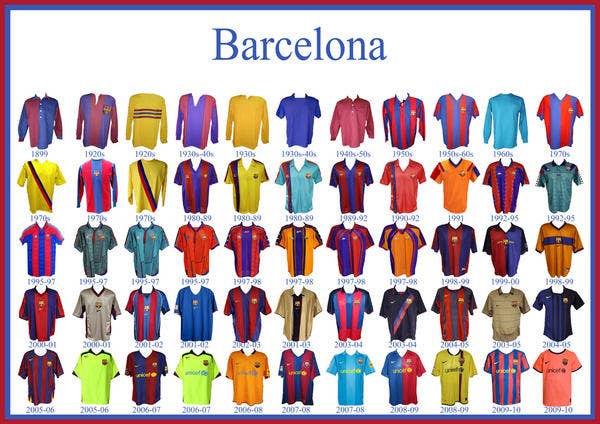The image showcases 55 different Barcelona Football Club jerseys arranged in 5 rows and 11 columns, each displaying various styles and designs. The background color is white with a red and blue border. At the top of the image, the word "Barcelona" is prominently displayed in blue letters beneath the title "Battle Longer." 

Examples of the detailed jersey designs include:
- The jersey on the top-left has long sleeves with a unique color split: blue on one sleeve and red on the other, while the body features a reversed color pattern with red on the left side and blue on the right.
- The jersey on the bottom-right has short sleeves, is predominantly orange, and features a Nike logo on the left chest, a printed name on the chest, and includes the year "2009-10" beneath it. 

The jerseys come in a variety of colors including red, purple, yellow, black, green, turquoise, brown, and orange, and feature both striped and solid patterns, illustrating the diverse range of designs available for fans and collectors.